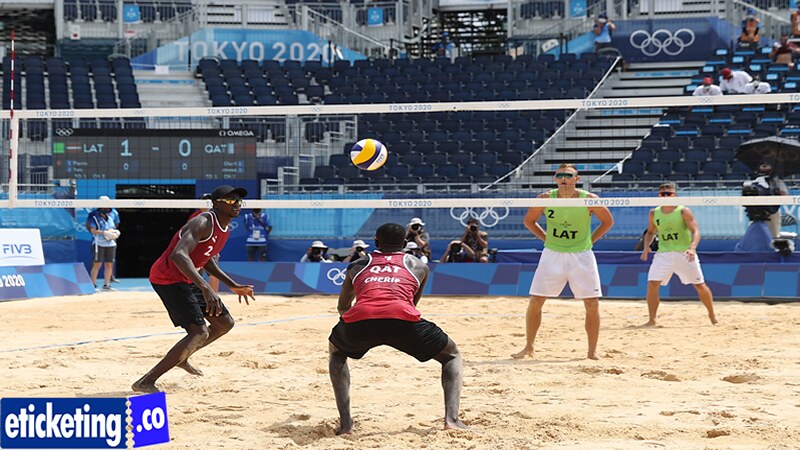The photograph captures an intense moment from a beach volleyball match during the Tokyo 2020 Olympic Games. The scene depicts two teams facing off on a sandy court, set against the backdrop of largely empty stadium stands. The team on the near side of the net consists of two dark-skinned male athletes from Qatar, both dressed in red tank tops and black shorts. One player, wearing a black baseball cap and sunglasses, is poised on the balls of his feet, ready for action. His teammate, also bent at the knee, is about to make a play on the volleyball suspended mid-air. 

Opposing them are two light-skinned male players from Latvia, identifiable by their green tank tops and white shorts with "LAT" emblazoned on them. Both Latvian players have blonde hair and wear sunglasses. The player closest to the net has his hands behind his back, signaling to his teammate, who stands slightly off-center, focused on the unfolding play. The scoreboard in the background shows a score of Latvia 1 and Qatar 0, hinting at the competitive nature of the match.

The photograph also includes various elements such as a volleyball net, numerous cameras, and sand, with the vibrant colors of the athletes' uniforms contrasting against the backdrop. Text within the image reads "Tokyo 2020" and "eticketing.co," anchoring the scene in its Olympic context.